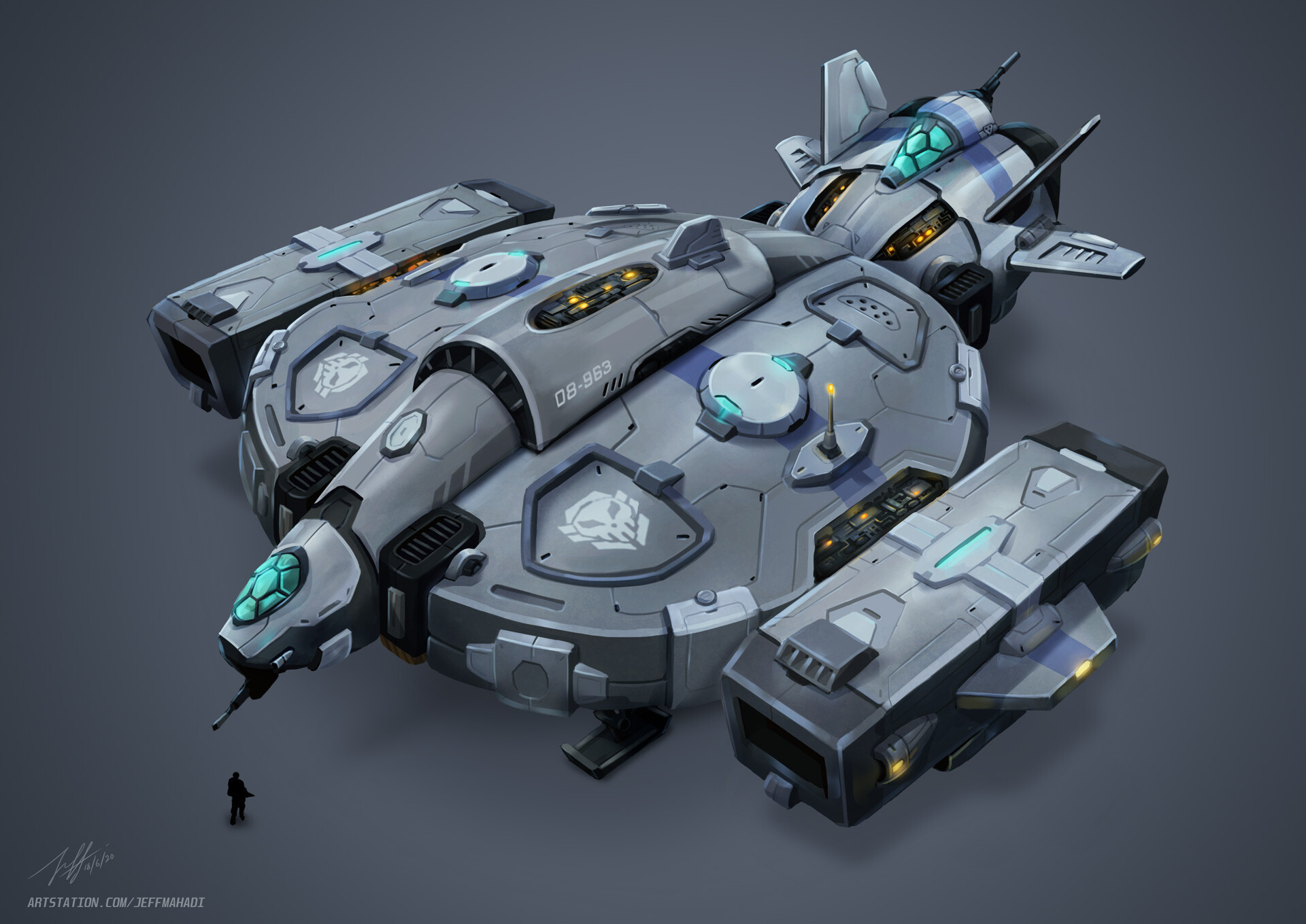The image showcases a digitally animated spaceship set against a flat, light gray background that subtly darkens towards the edges. In the bottom left corner, there is white text displaying a signature along with "ArtStation.com/Jeffrey Mahadi." Dominating the center of the image, the spaceship features a large, rounded central body with square-shaped wings extending on either side. The top of the ship has an antenna and an aqua emblem resembling a turtle shell, which also appears on the tail. The front of the ship, oriented towards the bottom left, has a prominent light green cockpit window and numerous light green lights. The tail end shows multiple metal fins and additional transparent windows with yellow lights. Notably, there are artistic details such as two skull designs near the wings and the number "08953" inscribed on the ship. To add scale, a small black silhouette of a person is seen standing under the spaceship, emphasizing the size and grandeur of this sci-fi craft.